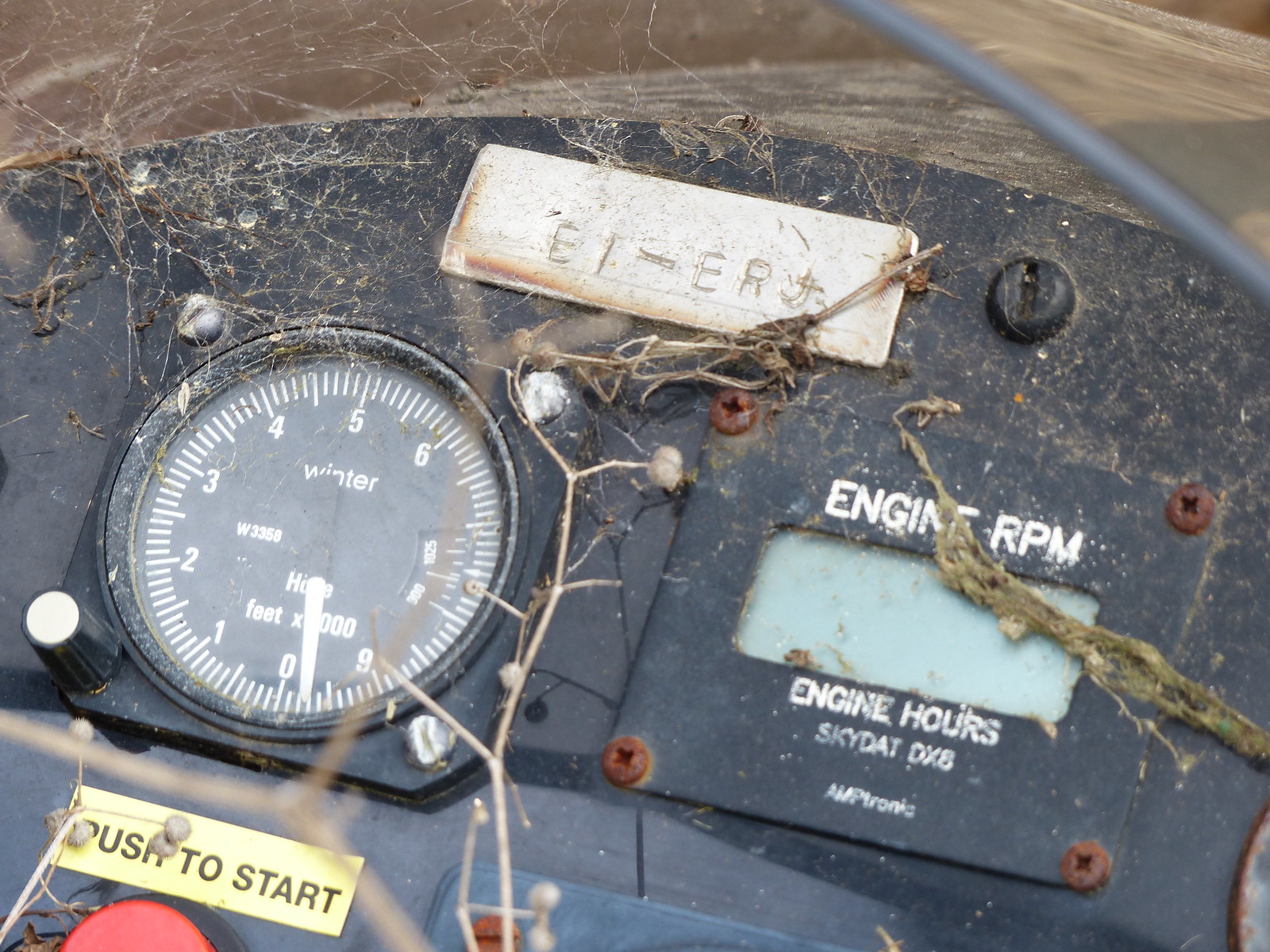The image is a detailed close-up of an old and weathered control panel, likely from an aircraft or similar machinery. The background is black, and the dashboard is cluttered with rusted bolts, screws, cobwebs, and debris, suggesting it has been abandoned for some time. Central to the panel, there’s a large meter labeled "winter W3350" that ranges from zero to nine. Another display marked "engine RPM" and "engine hours" with the brand "SkyDat DX6" is visible, surrounded by rusted bolts. A prominent feature is a red button at the bottom, highlighted with a yellow label that reads "push to start" in black lettering. An additional metal attachment at the top features the text "ELERJ." The whole assembly, beset with signs of age and neglect, appears to have been exposed to the elements, evident from the dirt, twigs, and cobwebs adorning it.